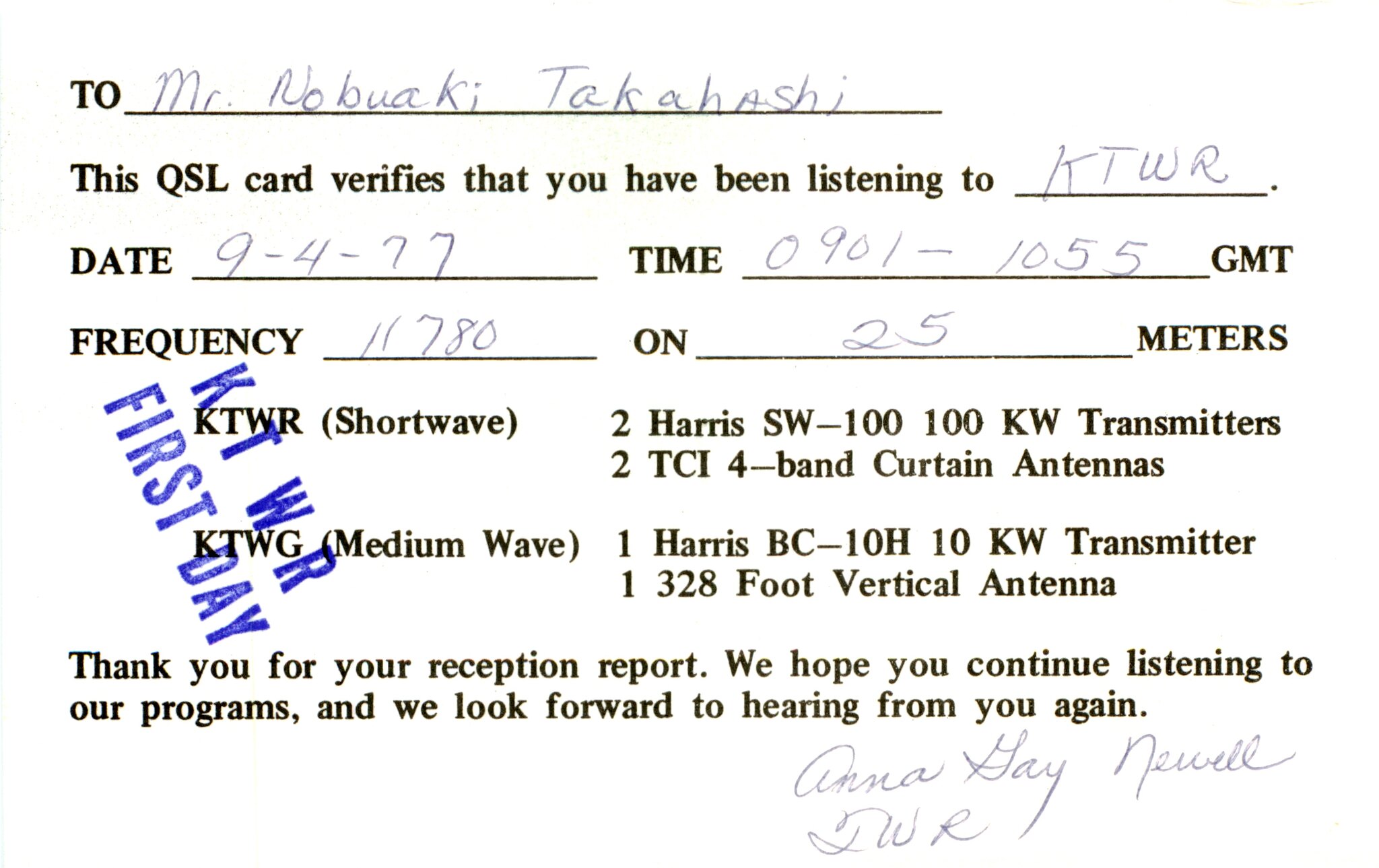This image is a detailed QSL card, a vintage print publication in landscape orientation, with a white background and black text. The card is filled out in pen and contains a blue stamp angled from the top left to the center, reading "KTWR First Day." Addressed to Mr. Nobuaki Takahashi, it verifies that he has been listening to KTWR shortwave radio. The card confirms reception on 9-4-77 from 09:01 to 10:55 GMT on the 11,780 kHz frequency at 25 meters. The technical details specify the use of 2 Harris SW-100 100 KW transmitters and 2 TCI 4-band curtain antennas for shortwave, as well as 1 Harris BC-10H 10 KW transmitter and a 3,280-foot vertical antenna for medium wave. The card concludes with a message: "Thank you for your reception report. We hope you continue listening to our programs, and we look forward to hearing from you again," signed in ink by Anna Gay Newell, TWR.